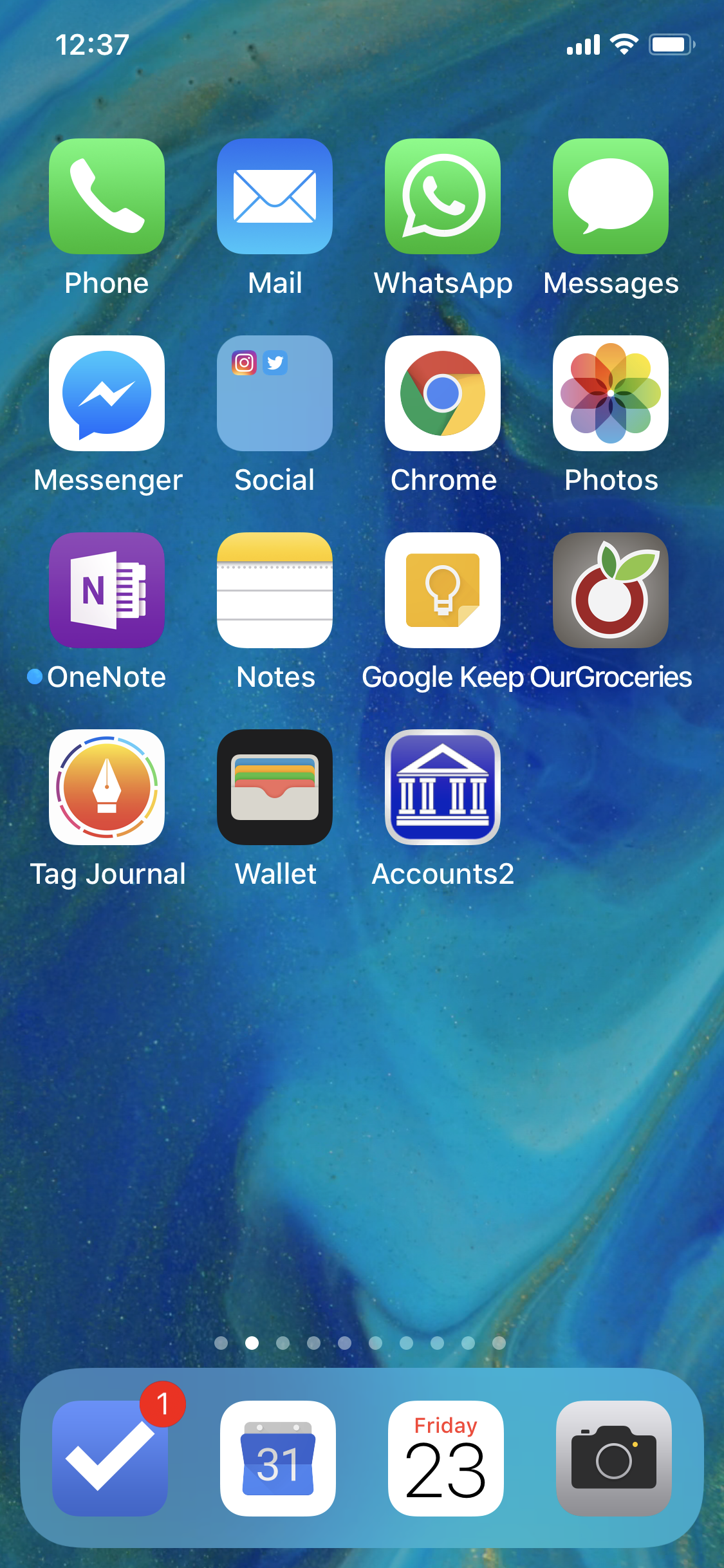Screenshot of an iPhone Home Screen:

The image showcases the home screen of an iPhone, displaying various app icons arranged in a structured layout. Starting from the top row, from left to right, the first icon is the "Phone" app, a green icon with a white phone receiver. Next to it is the "Mail" app, depicted as a blue envelope. Continuing right, the "WhatsApp" icon is visible, represented by a green speech bubble with a white phone symbol inside. Following this is the "Messages" app icon, a green speech bubble.

In the second row, from left to right, the first icon is "Messenger," identified by a blue speech bubble with a white lightning bolt. Adjacent to it is a folder labeled "Social," containing icons for "Instagram" (a colorful camera) and "Twitter" (a blue bird). Next in line is the "Chrome" browser icon, a colorful circle with a blue center. Finally in this row, there is the "Photos" app, depicted by a multicolored flower.

On the third row down, from left to right, the first icon is "OneNote," represented by a purple square with a white "N," with a blue dot indicating a notification or update. Following this is the "Notes" app, a yellow and white notepad. Next is the "Google Keep" icon, a lightbulb on a yellow background. The last icon in this row is "Our Groceries," distinguished by a brown paper bag filled with groceries.

The fourth and final row features, from left to right, the "Tag Journal" icon (not visibly detailed but likely a journaling app), "Wallet" icon (black with a white wallet graphic), and the "Accounts" icon, possibly representing financial tracking or management (details are unclear).

At the bottom of the screen, in a light blue bar known as the dock, there are four icons: from left to right, a "Check Mark" icon (likely a to-do list or task manager), the "31" icon (possibly a calendar app), the "Calendar" app (white with a red header and dates displayed), and the "Camera" app, a grey camera lens.